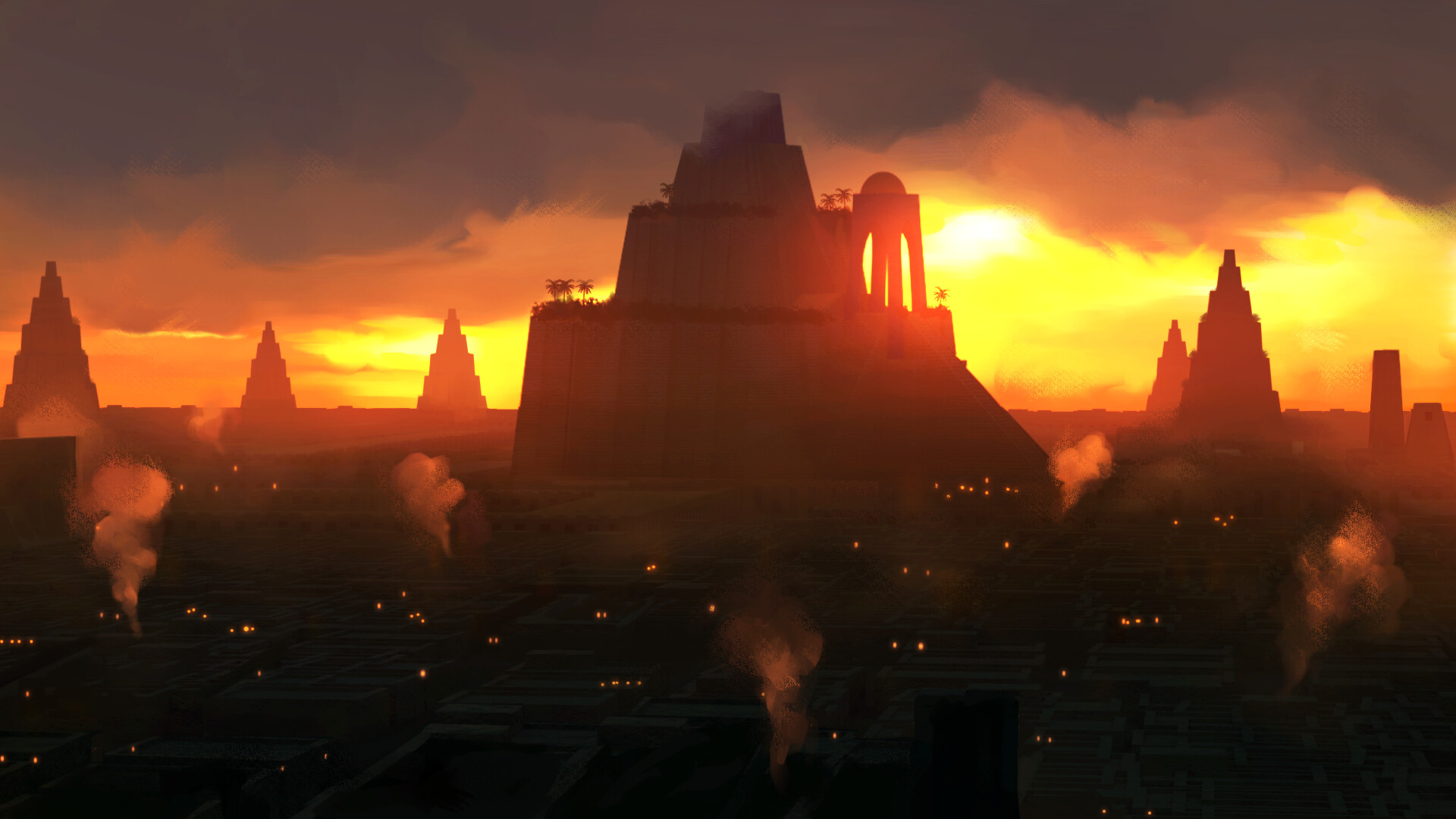The image depicts a city skyline enveloped in a thick, smoky haze, giving it an eerie, almost film-like quality. Dominating the scene is a large central building, surrounded by numerous smaller structures, many of which have step-pyramid-like tops. Wisps of white smoke rise from various smokestacks, contributing to the heavy, smoke-laden atmosphere. The sky is a muted mixture of amber, orange, and blackish hues, with the setting sun barely visible through the dense smoke, casting a yellowish glow over the entire scene. Scattered lights in some windows provide the only illumination in this otherwise shadowy, dystopian landscape, which bears a striking resemblance to a movie set.